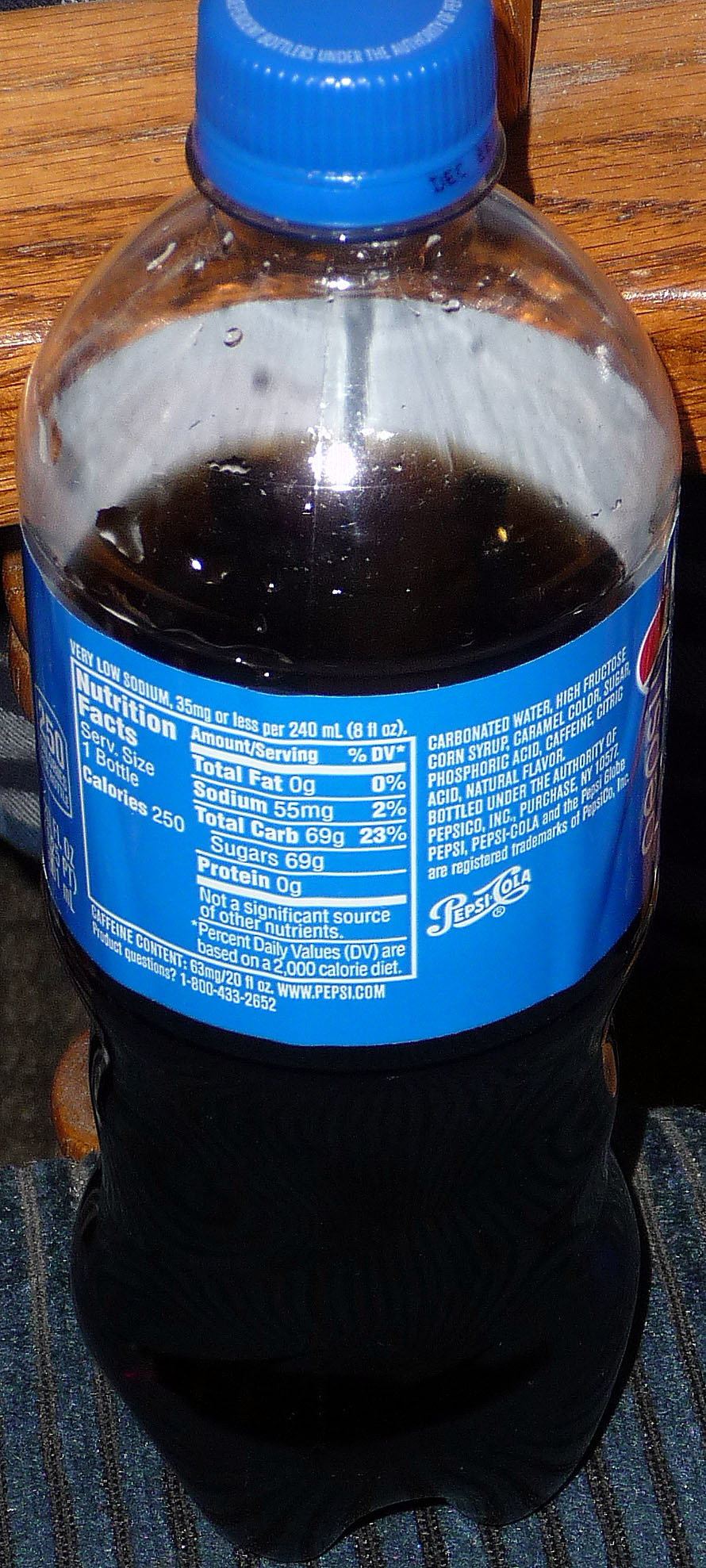This image features a close-up of a Pepsi soft drink bottle. The bottle, made of clear plastic, has a light blue plastic cap. Inside, the bottle contains a dark cola drink and appears to be about two-thirds full. It is placed on a placemat with alternating blue and brown stripes, resting on a brown table. In the background, there's a wood-grained wall, contributing to a rustic ambiance. A light source shines brightly on the bottle, causing reflections on its surface. Though the front label isn't fully visible, the side of the label prominently displays the "Pepsi Cola" logo and nutritional information.